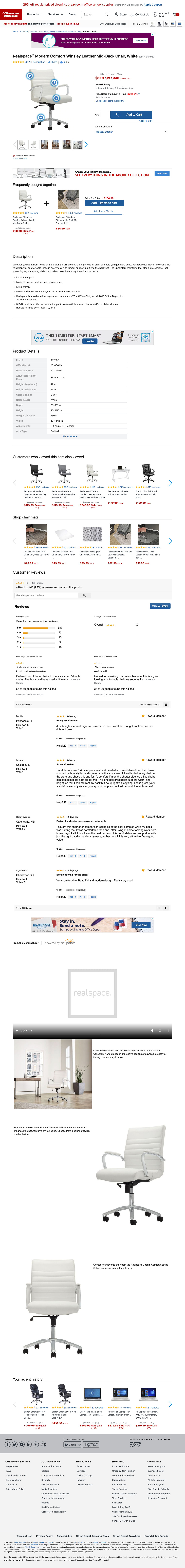This image consists of three distinct screenshots, illustrating the process of purchasing a white office chair. Each screenshot appears to be part of an online product listing, though the exact company is not identifiable due to the cluttered presentation. 

In the first screenshot, the image depicts the ergonomic features of the chair, detailing the adjustable components such as the legs and various support mechanisms necessary for comfort. The accompanying text, which should describe these features, is overly compressed and difficult to read, adding to the visual confusion.

The second screenshot overwhelms the viewer with an excessive amount of text in various colors—black, red, and blue—particularly red, causing further disorganization and obscuring the price and other critical details about the chair.

The third screenshot presents alternative options, showcasing five other office chairs based on the search criteria. This section eventually leads to an image of the featured chair in a usage context—a staged setting intended to show the chair in an office or living space. The setting includes a desk to the left and a window with a plant to the right, all placed on a wooden floor. However, the overall layout is poorly executed, making it challenging to clearly understand the advertisement's origin and purpose.